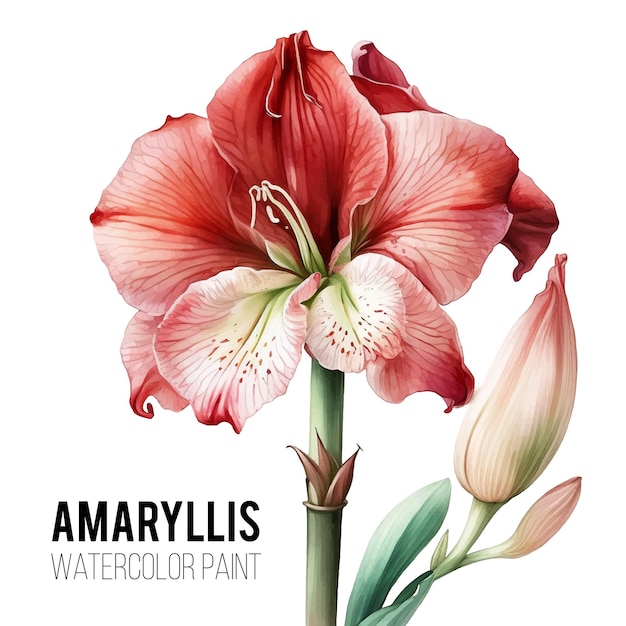The image features a meticulously detailed watercolor painting of an amaryllis flower against a white background. The top left corner displays the word "AMARYLLIS" in boldface font, while beneath it, in a thinner style, are the words "WATERCOLOR PAINT," both rendered in all caps. The central focus is a stunningly realistic amaryllis, reminiscent of a classical botanical illustration, capturing every intricate detail from the veins to the stamen and stem. The main bloom, prominently situated, showcases a rich red color with hints of brown. Two of its front petals are speckled and tipped with white. To the right, two additional blooms are depicted in various stages of development. The yellow-green stem features three small leaves, complemented by two more blue-green leaves positioned beneath the blossoms. The exquisite shading and delicate linework highlight the dedication and skill invested in this formal and elegant artwork.